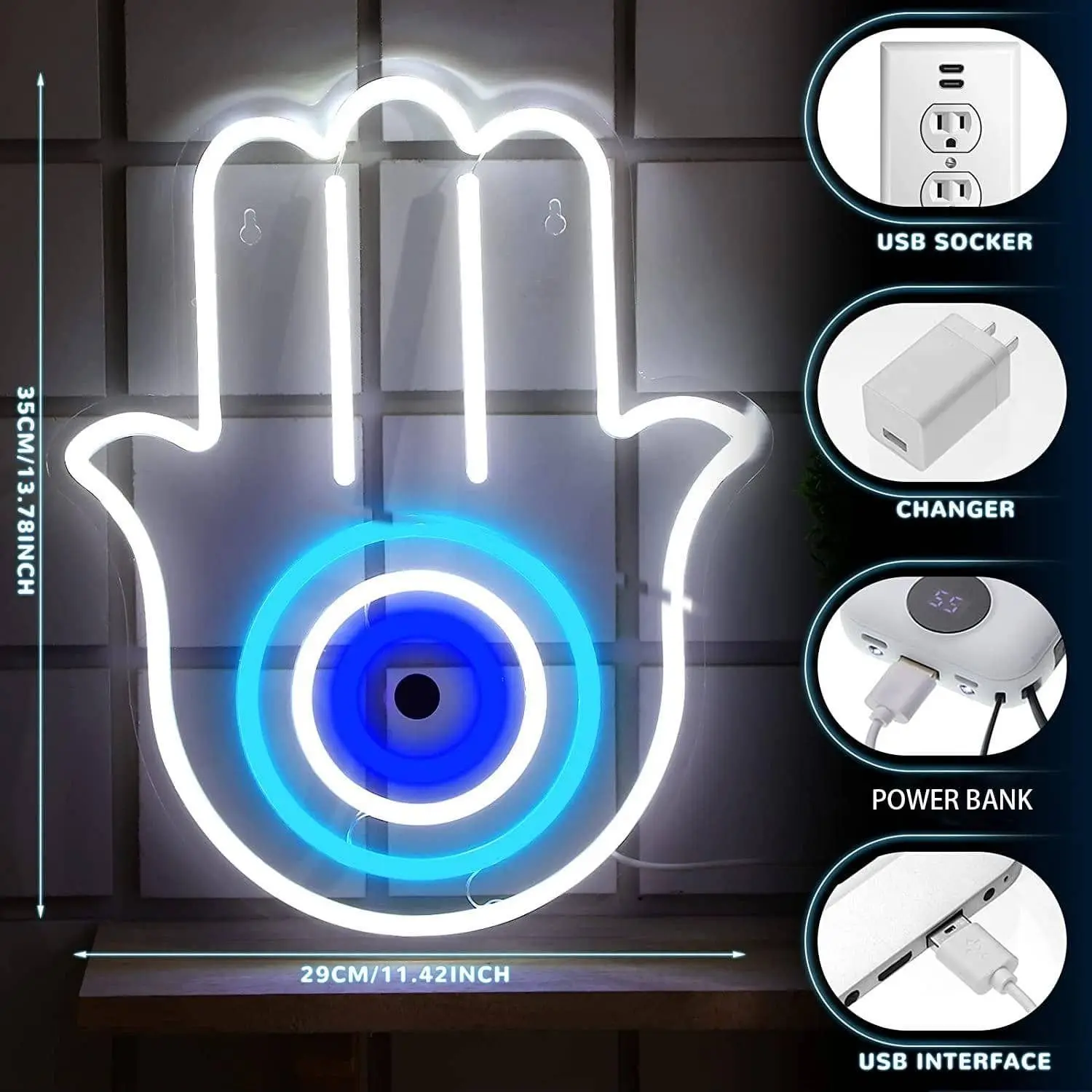The advertisement features a unique light fixture designed as a hand with an eye at its center, resembling a neon sign. The hand, outlined in glowing white lights, has its thumb and pinky outstretched while the three middle fingers are pointed upwards. The eye in the center of the hand consists of three concentric circles in light blue, white, and dark blue, with a black dot at its center, suggestive of a protective symbol. The fixture is displayed on a wooden table against a backdrop of white tiling, with its lights turned on to showcase its vibrant glow.

To the right of the image are four stacked ovals, each highlighting the fixture’s power options with corresponding pictures: a USB socket, a charger, a power bank, and a USB interface. Additionally, measurements on the side indicate the product dimensions as 35 cm / 13.78 inches in height and 29 cm / 11.42 inches in width, providing potential buyers with a clear understanding of its size.

Overall, this detailed representation emphasizes the artistic design, power versatility, and dimensions of the light fixture, making it an intriguing and practical purchase option.